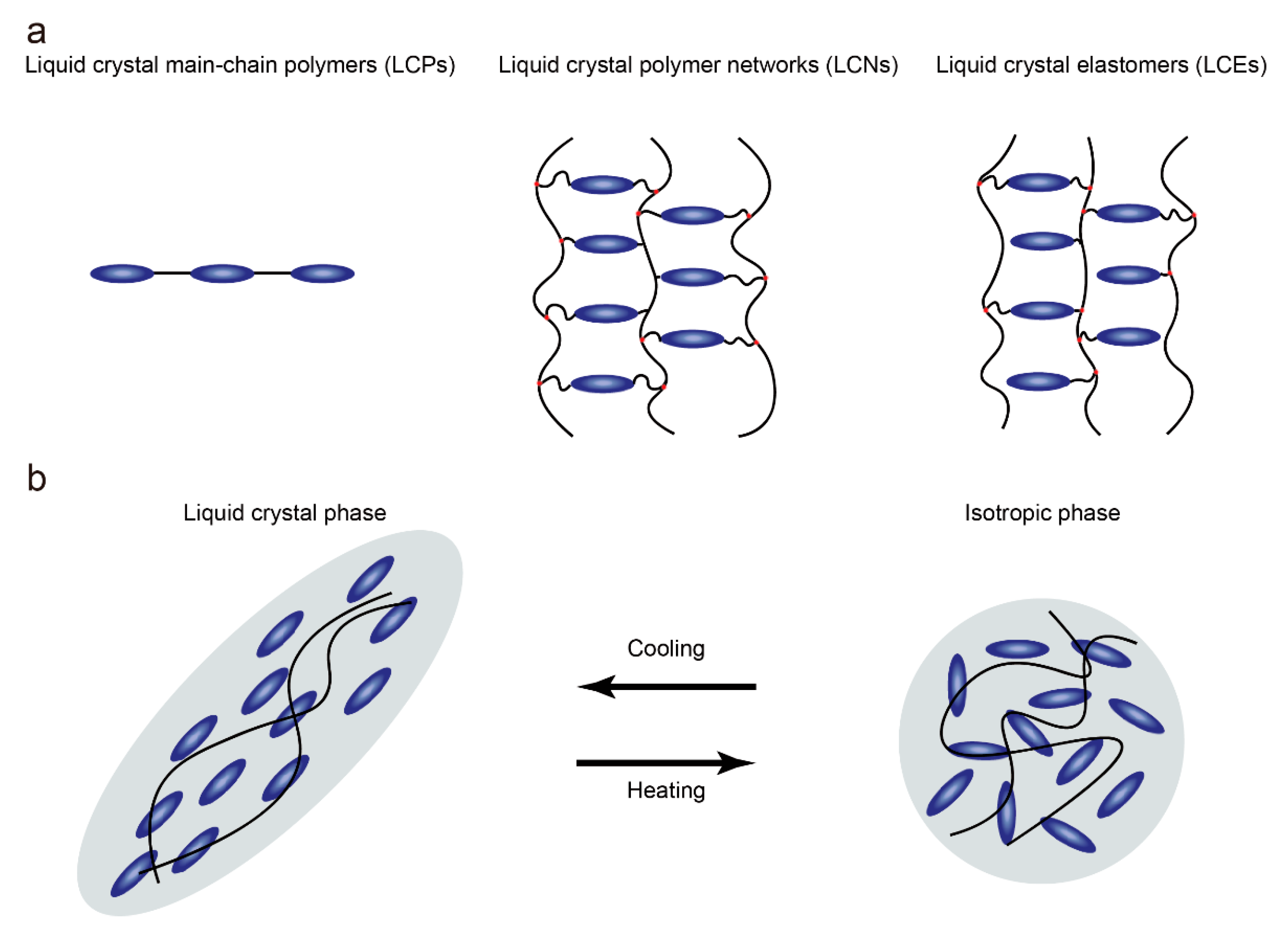The diagram is divided into two parts, labeled A and B, set against a white background. Part A showcases three different configurations of liquid crystal polymers. On the left, it illustrates "Liquid Crystal Main Chain Polymers (LCPs)" with blue oval shapes connected in a linear fashion by black lines. The middle section features "Liquid Crystal Polymer Networks (LCNs)," represented with the blue ovals arranged on what looks like a rope ladder, with four ovals on the left and three on the right, all connected by squiggly black lines. On the right, it shows "Liquid Crystal Elastomers (LCEs)," which are similar to the LCNs but with somewhat straighter sides. Part B depicts a transition diagram of the liquid crystal phase. On the left, labeled "Liquid Crystal Phase," it has black arrows pointing left to "cooling" and right to "heating," leading to the right side labeled "Isotropic Phase." Both phases are represented by blue ovals and squiggly lines.